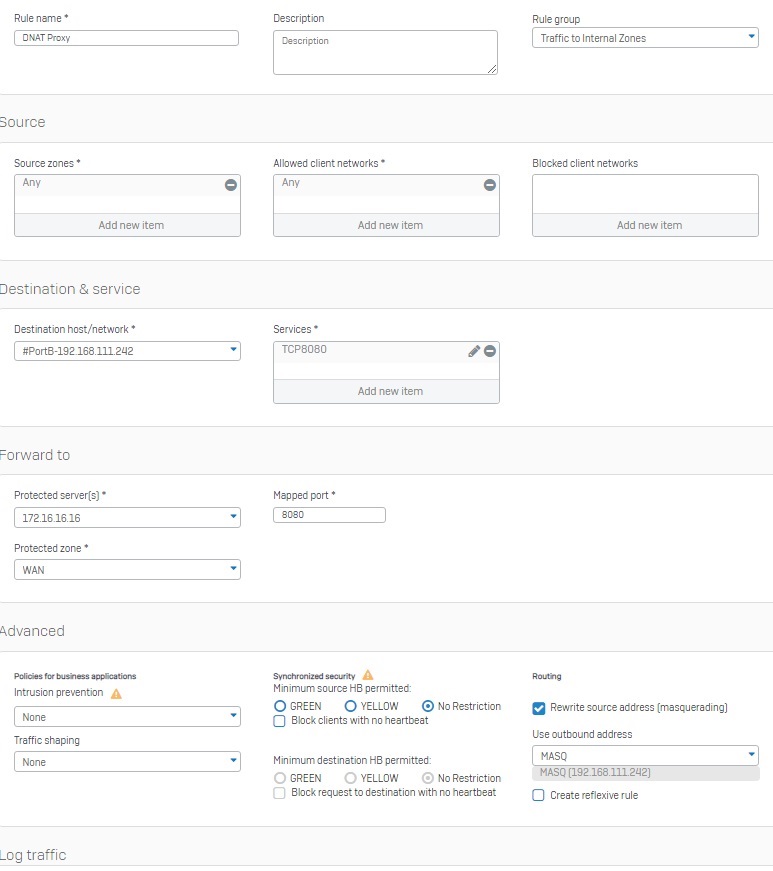The image displays a screenshot of a network configuration interface featuring various input fields and settings. At the top, the "Rule Name" is specified as "DNAT proxy." In the "Description" field, it simply says "description." The rule group is labeled "Traffic to Internal Zones."

Further down, under the "Source" section, it shows "Source Zones" set to "any," "Allowed Client Networks" also set to "any," and "Blocked Client Networks" with an option to "add new item."

In the "Destination and Service" section, it provides an area for "Services" with an option to "add new item." Additionally, it includes fields labeled "Destination Host/Network," "Forward To," where it lists "Protected Servers," "Protected Zone," and "Mapped Port."

The "Advanced" section features settings for "Policies for Business Applications" and "Intrusion Prevention." An exclamation point inside a triangle indicates some form of alert or warning. Under this, it specifies "None" for both, and "Traffic Shaping" is set to "none." The "Synchronized Security" section shows options for "Minimum Source HB permitted," color-coded indicators for "Green," "Yellow," "No Restriction," and settings for "Blocked Clients with no Heartbeat."

At the bottom of the interface, there's an option labeled "Log Traffic."